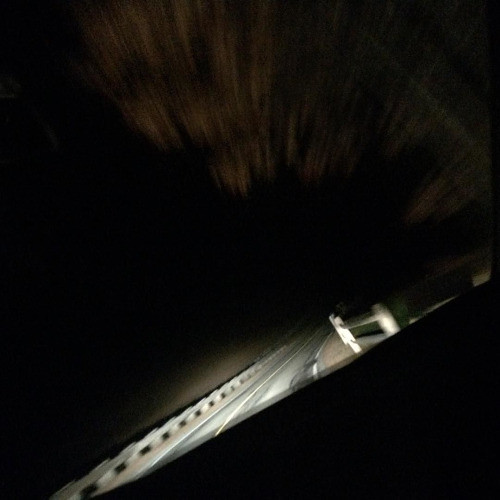A nighttime photograph captures the motion of trees as they blur past, suggesting it was taken from a moving vehicle. The sky is an inky black, with the only illumination coming from a bright light, possibly a car's headlight. The road ahead is gray with a distinct white stripe down the middle, flanked by short, gray guardrails. To the right, a white picket fence runs parallel to the road, adding a quaint touch to the scene. The tallest tree near the vehicle appears greenish-brown, although the entire image is quite blurry, emphasizing the swift movement when the photo was taken.